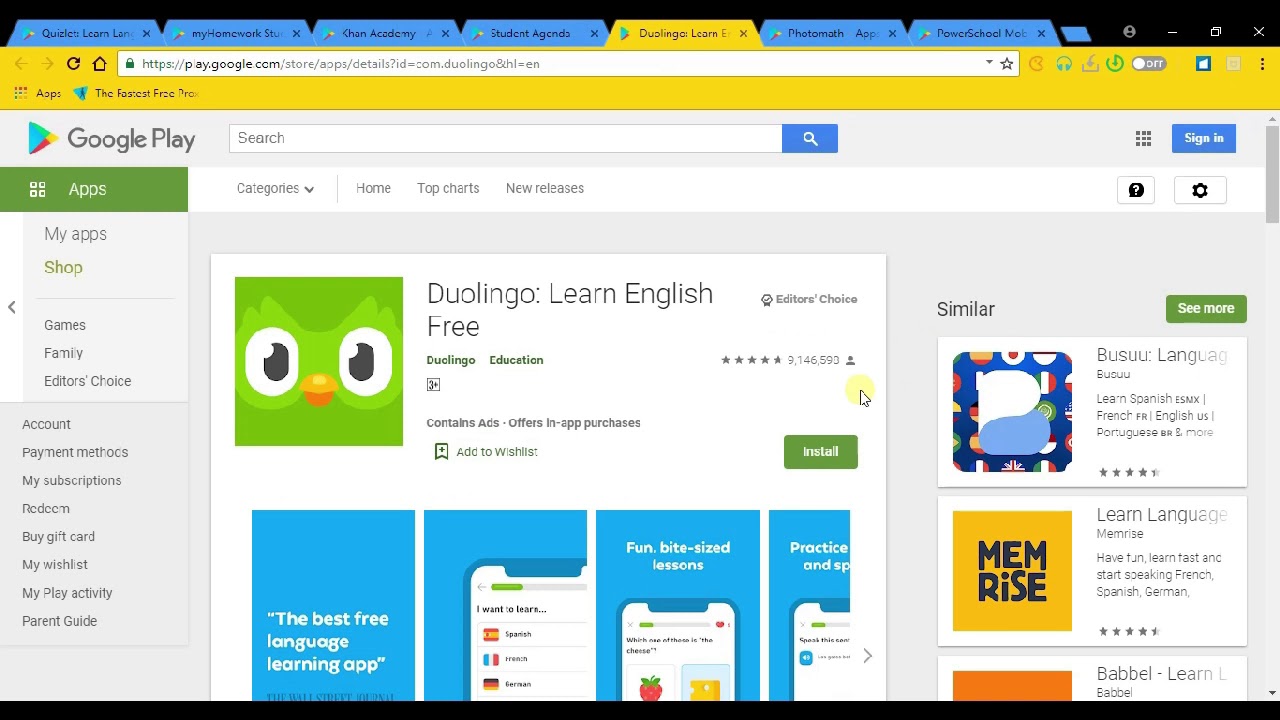This image showcases the Google Play Store interface as viewed on a mobile device. At the top of the screen, there are eight tabs offering navigation options. The central focus of the screen is the Duolingo app, highlighted with its distinctive green bird logo and accompanied by the app's name. Beside it, there is a prominent blue button inviting users to sign in. The Google Play Store is presented in its iconic color scheme of blue and red. On the left side, various other application icons are displayed, representing different categories and options for users. At the bottom of the screen, a preview section provides a glimpse into the Duolingo app's features and functionalities. All these elements come together to form a comprehensive and user-friendly interface for exploring and downloading apps.